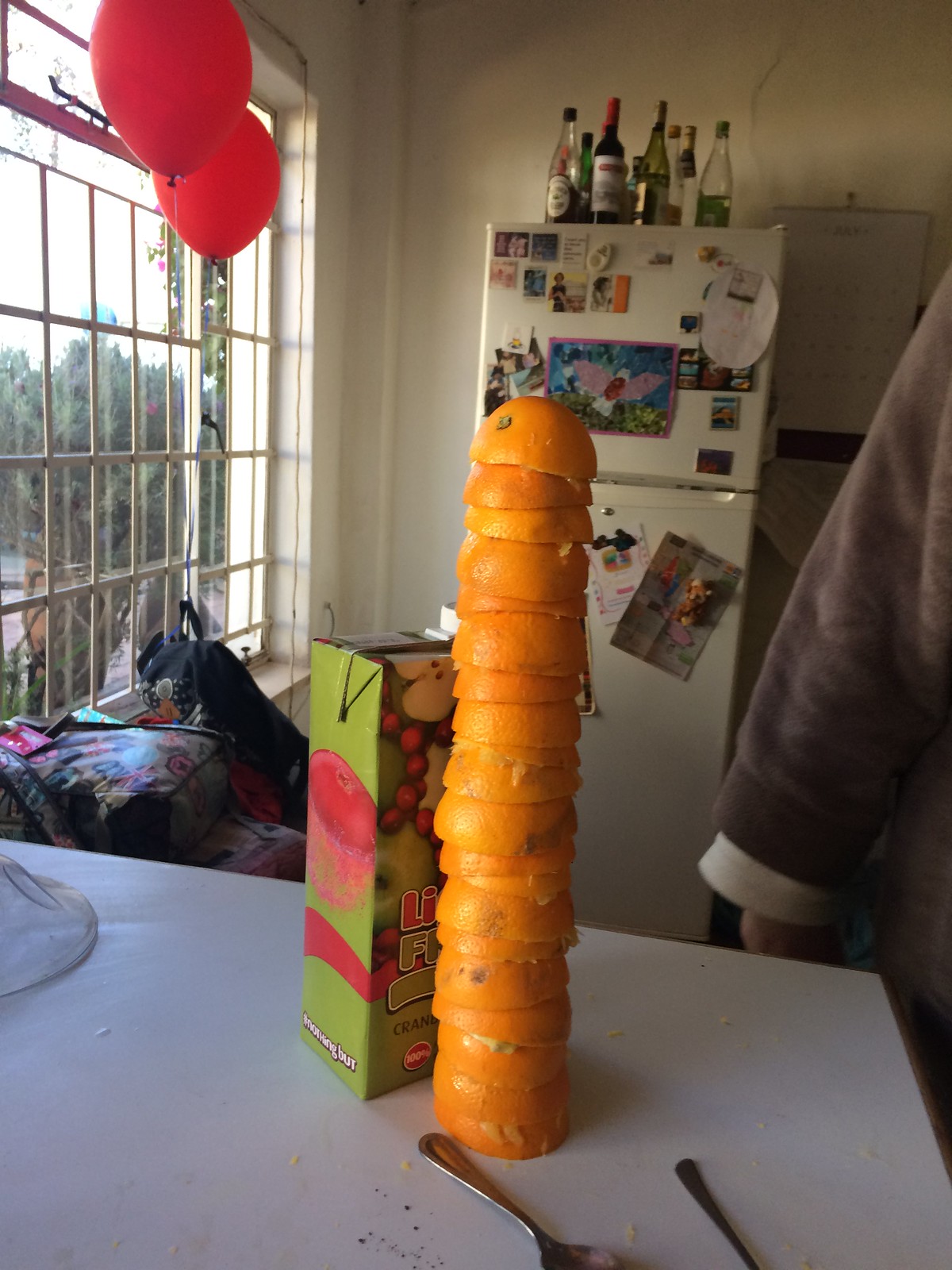This vibrant color photograph captures a bustling kitchen scene, richly detailed with various elements. Dominating the foreground is a remarkable tower of hollowed-out orange peels, meticulously stacked, suggesting they were likely juiced. This tower, composed of approximately 20 halves, reaches an impressive height and sits on a white table, which is littered with some crumbs and black specks. Just beside the tower, there is a green carton, possibly juice, adorned with pink lips and some unreadable text that might be in an Asian script. Two pieces of silver cutlery, likely a spoon and another utensil, lie in front of it.

In the background, a white refrigerator is covered in colorful magnets and children's artwork, including a childlike painting of a bird. The fridge is topped with numerous bottles, possibly wine, adding to the kitchen's lived-in feel. To the left of the fridge stands a large window, draped with a multi-colored throw on its bottom half. Beyond the window, you can glimpse trees and vegetation outside, while inside, two red helium balloons float near the top. In the corner of the image, a person's grey jacket with white edging can be seen. Completing this detailed scene are some book bags placed near the window, adding to the sense of an active household.